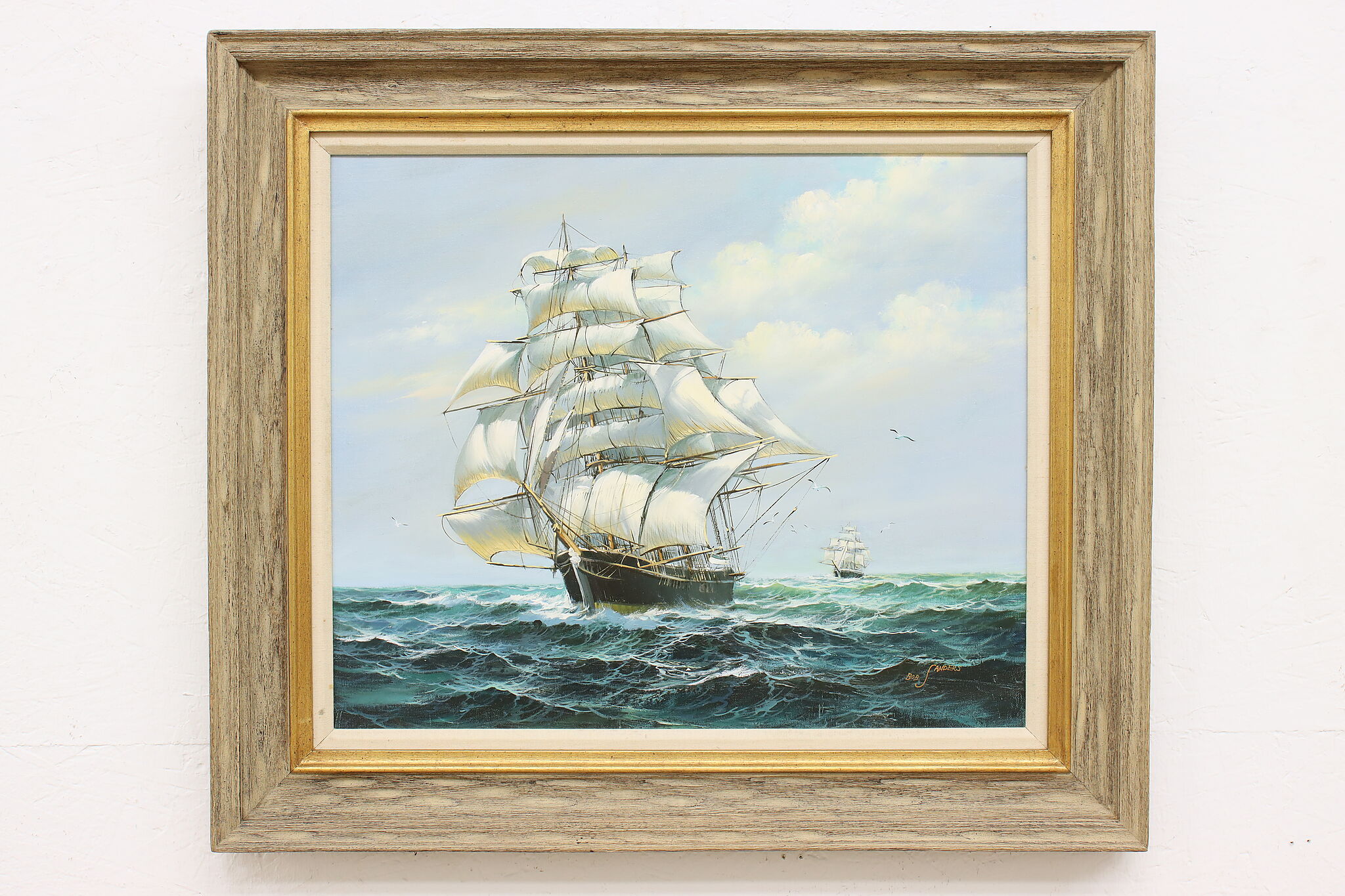This image depicts an oil painting of a majestic ship navigating through turbulent ocean waves. The painting, housed in a wide vertical rectangular frame, features a light brown wood outer frame with additional gold and white borders. The scene captures a vivid light blue sky adorned with white puffy clouds, contrasting against the darker foreground of the stormy green and blue ocean, which is accentuated with white-crested waves. Dominating the center of the painting is a grand, dark-colored ship leaning slightly to the left, its towering masts adorned with numerous white sails that have subtle yellow highlights at their bases. In the deep background, another similar ship sails upright, adding depth to the composition. The dynamic nature of the sea is emphasized by the roughness of the waves, while seagulls can be spotted to the right of the main ship, providing a touch of life and movement to the scene. The painting's rich palette includes hues of dark and light green, blue, off-white, tan, beige, brown, black, and gold, all meticulously blended to convey the artist's skill and attention to detail. This visually striking artwork hangs against a light gray wall, inviting viewers to immerse themselves in its historical maritime narrative.